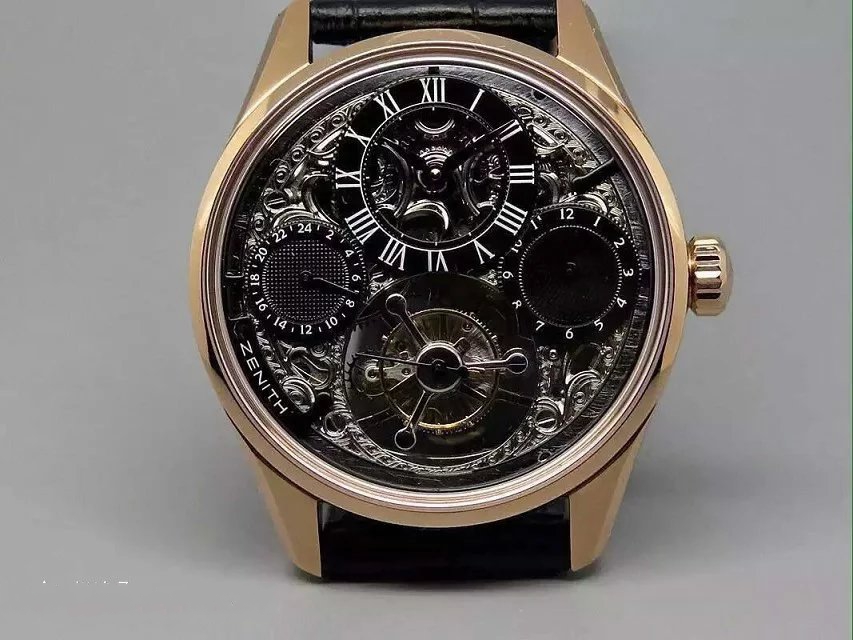This detailed close-up photograph captures an exquisite Zenith watch. The watch prominently features a sleek black leather strap and a blackened gold or brass casing, exuding a sophisticated allure. The face of the watch is adorned with gold and showcases several intricately designed sub-dials. The main dial displays the time with Roman numerals, while two smaller sub-dials, presumably a 24-hour and a 12-hour clock, flank the left and right sides. An additional sub-dial with multiple hands sits below the center.

Notably, the branding "ZENITH" is clearly visible in capital white letters positioned towards the 7-8 o’clock area on the watch face. The overall dial design appears gray, complemented by the exposed mechanical elements behind the watch faces, offering a glimpse into the precise craftsmanship. The watch’s time indicates it is approximately 10:10. The background of the image is gray, with a small white mark on the bottom left corner. All these elements collectively highlight the intricate details and luxurious quality of the Zenith watch.